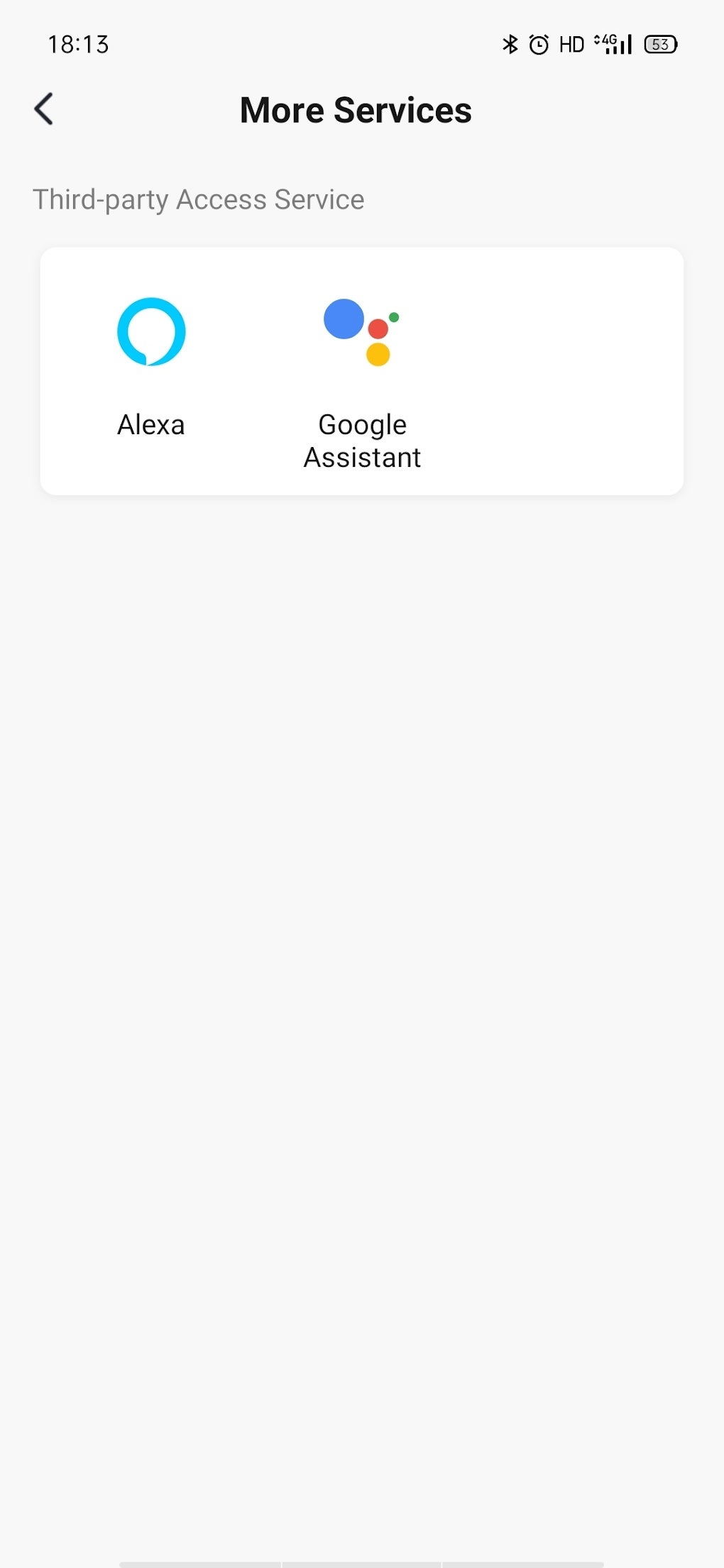The image is a screenshot of a smartphone interface. The background is predominantly gray, with a white rectangle at the top. In the upper left corner, the time is displayed as 18:13 in black text. To the upper right, various icons are visible, including the Bluetooth icon, an alarm icon, the letters "HD," reception bars, and a battery icon.

Beneath the status icons, the interface shows a black left-pointing arrow. Centrally, bold black text reads "More Surfaces," and below that, in gray text, it says "Third-Party Access Service."

Within the white rectangle, there are two icons. The first icon on the left is for Alexa, featuring the word "Alexa" in black accompanied by a circular blue brush stroke oriented clockwise. The second icon, to the right, is for Google Assistant, with "Google Assistant" in black text and the corresponding icon of four dots in the colors red, blue, green, and yellow.

The remainder of the screen is blank gray space.